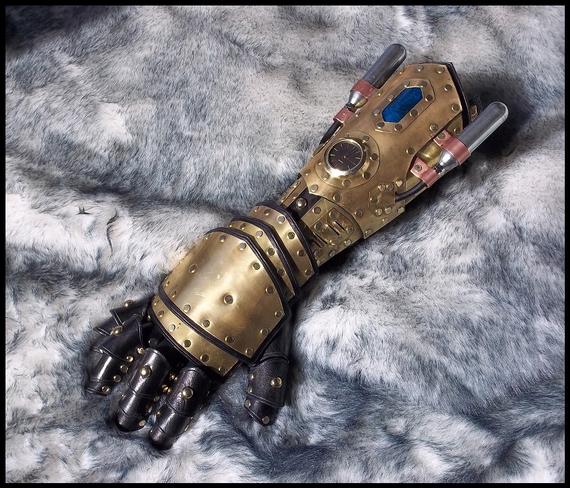The image features a meticulously crafted medieval-style armored glove set against a luxurious faux fur fabric with white, gray, and black hues. The armor's design is a striking blend of dark granite for the fingers and lustrous gold for the wrist and arm sections, each piece riveted and soldered together to allow flexibility. A prominent feature is the embedded timepiece at the wrist, which adds a steampunk flair, complemented by blue jewels and black accents. Pink bands and small cartridge-like details, possibly resembling nitrous oxide holders, adorn the glove, enhancing its intricate and sturdy appearance. The entire setup exudes a staged, yet visually captivating aesthetic, making it seem like a blend of historical and fantastical elements.